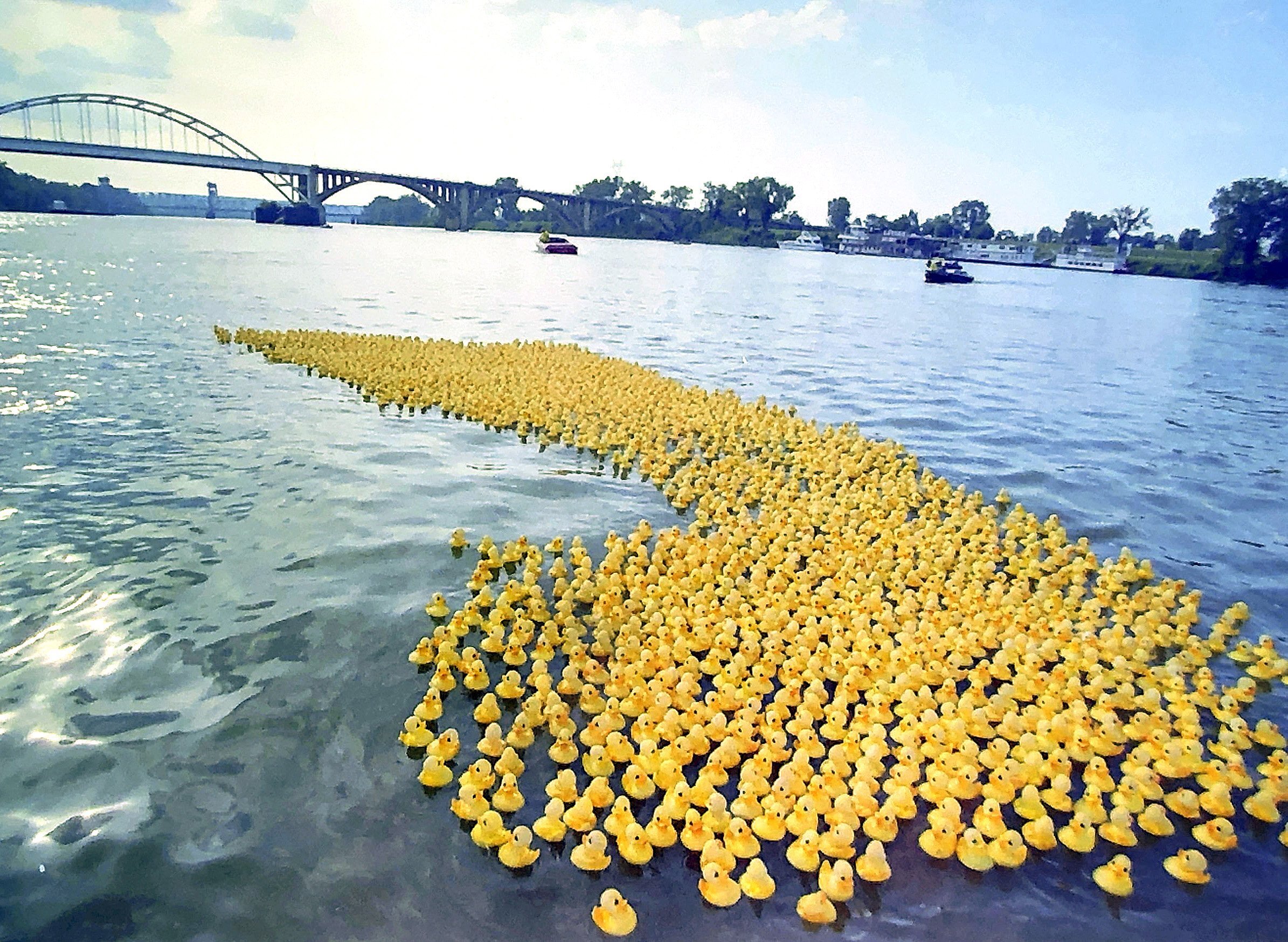In this captivating image, a major river is the setting for a whimsical scene that immediately captures attention: the water's surface is covered with hundreds of little yellow rubber ducks, clustered together, likely participating in a rubber duck race. In the foreground, these cheerful ducks create a lively spectacle as they float atop the river. Behind this vibrant crowd, two small boats can be seen navigating the water, while further in the distance, more boats are docked by the land. The landscape around the river is lush with greenery and trees, adding natural beauty to the scene. A large bridge spans across the river from the right side to the left, combining elements of cement and steel, indicating possible renovations. The sky above is a striking mix of clear blue and patches of white clouds, contributing to the overall picturesque and slightly hazy atmosphere. Off to the right, there are buildings peeking through, but the main focus remains the delightful swarm of rubber ducks dominating the river's surface.